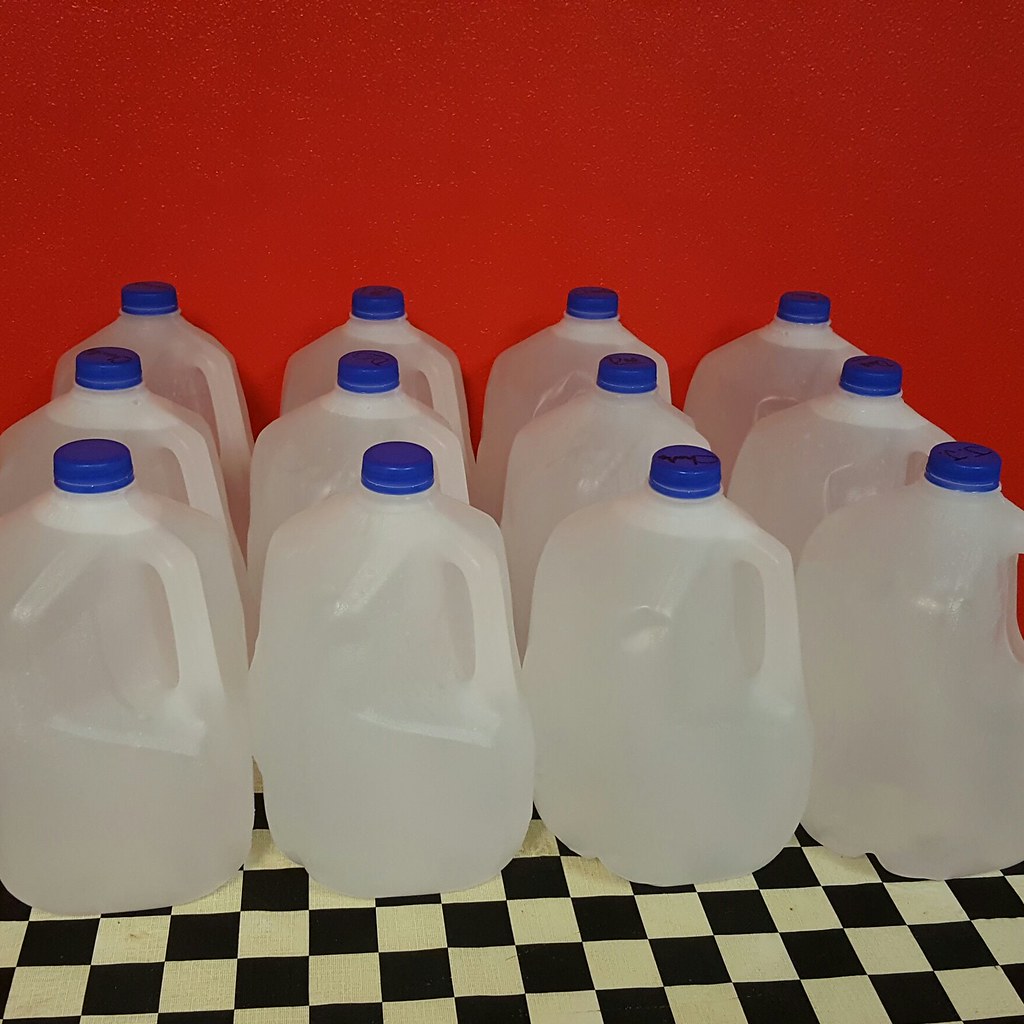This detailed photograph depicts 12 nearly identical clear plastic gallon jugs of water, each sealed with a blue twist-off cap, arranged meticulously in three rows of four on an old, slightly dingy black and off-white checkerboard floor. The jugs are positioned with their handles diagonally to the right, in front of a plain, vivid red wall. The jugs are almost completely full, with eight of them displaying small air pockets beneath the cap, while four are filled to the brim without any visible air space. Several jugs show minor side dents but remain otherwise intact. Notably, a thin hairline gap around the safety ring on each cap suggests they have been opened before. Shadows cast by the jugs and their alignment give the scene a somewhat symmetrical and orderly appearance.